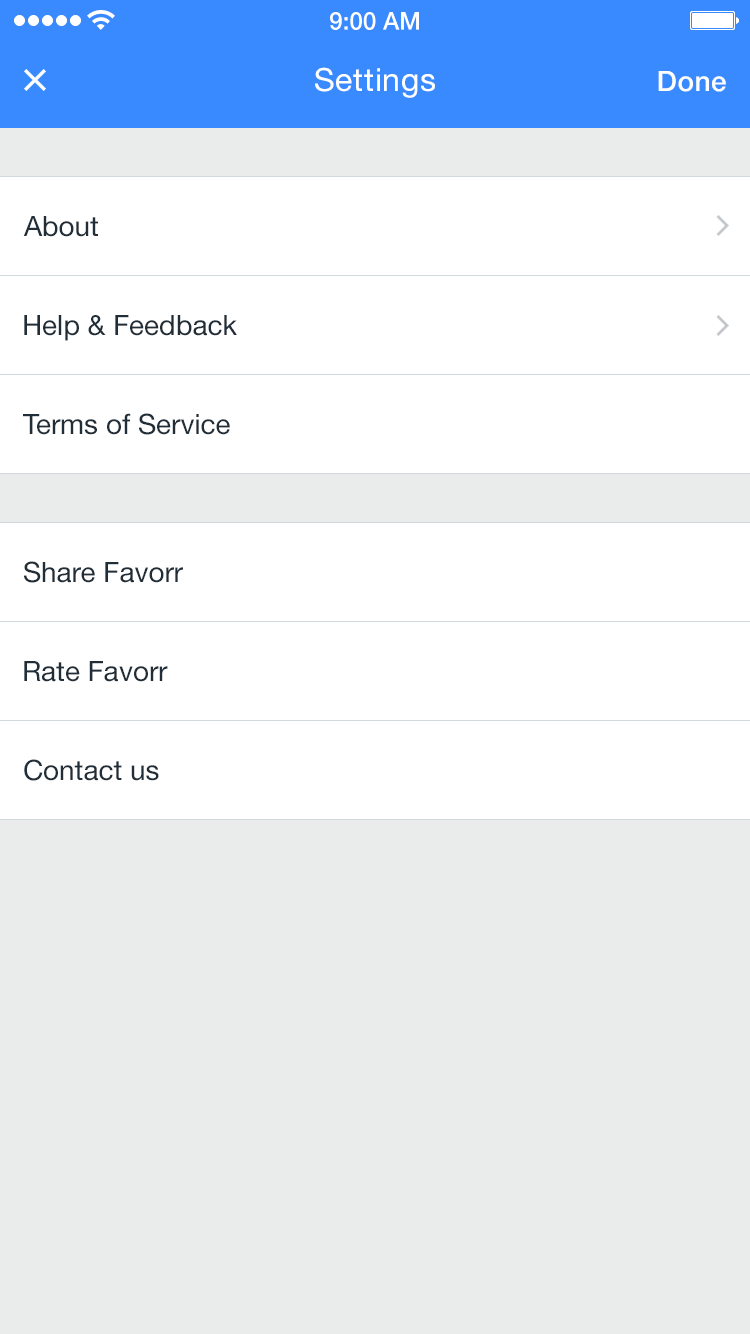Screenshot of a Mobile Phone Settings Page

The image displays a screenshot of a mobile phone's settings page, likely from an iPhone given the interface design. At the top, the screen shows a blue status bar indicating full signal strength with five dots and maximized Wi-Fi connectivity. The time is displayed as 9 a.m., and the battery icon on the top right corner indicates a full charge.

Within the main view, the screen presents a header with an "X" to close the settings menu and text options labeled "Settings" and "Done." Below the header, the primary settings options are listed:

1. **About:** An expandable menu indicated by an arrow.
2. **Help and Feedback:** Another expandable menu with a similar arrow indicator.
3. **Terms of Service:** This appears as a standard clickable link.

A gray divider separates these primary options from additional ones below:

4. **Share Favor**
5. **Rate Favor**
6. **Contact Us**

These additional options are clickable and likely open new windows or links for further interaction. At the bottom of the screen, there is a light gray text box, presumably for users to input information when contacting support. Although not visible in the screenshot, it is implied that there is a "Submit" button associated with this input field for sending the message.